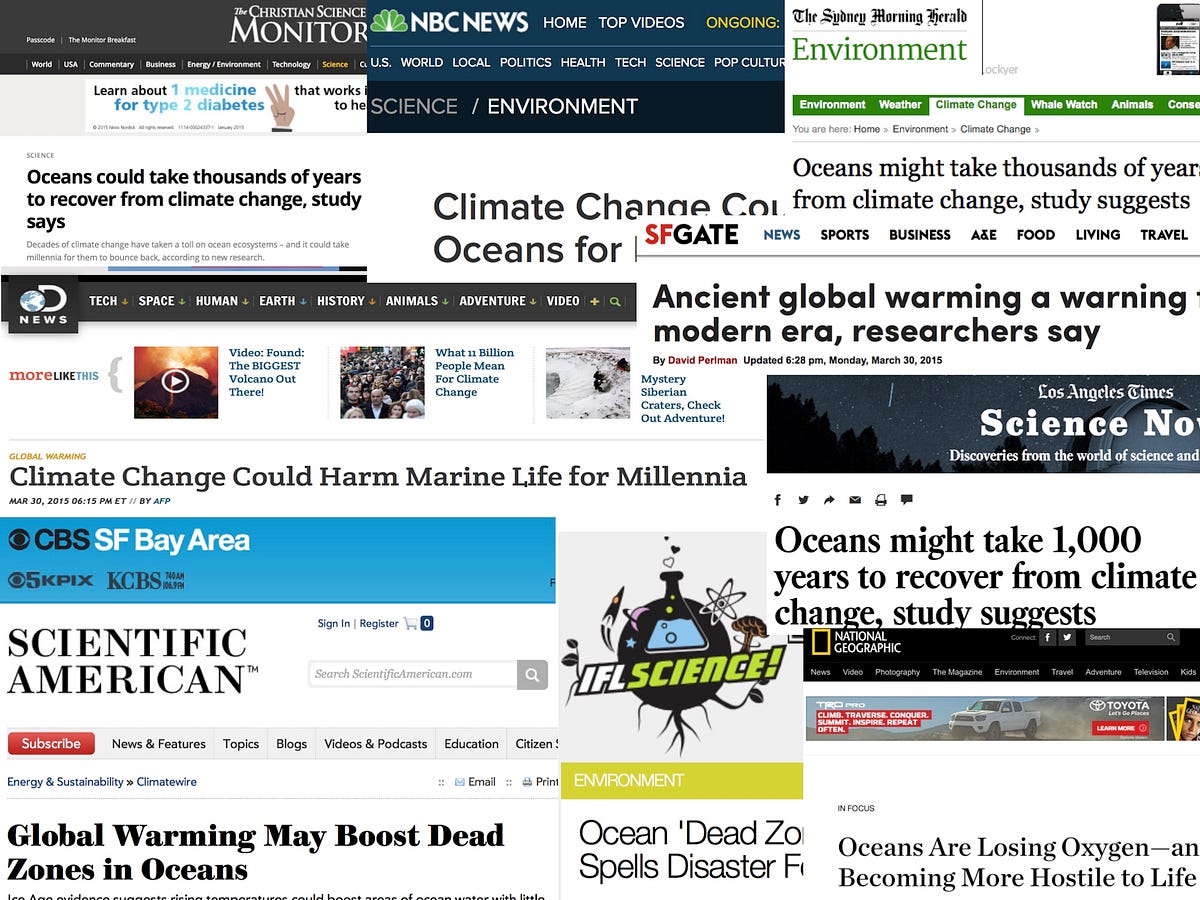A large, square collage of various environmental and science headlines extensively covering climate change and its effects on oceans. The top-left section features a portion of the Christian Science Monitor webpage, partially overlaid with the NBC News logo and menu options like "Home," "Top," "Videos," and "Ongoing." Adjacent on the right, headlines from the Sydney Morning Herald's environment section prominently highlight climate change. Below, an article states, "Oceans could take thousands of years to recover from climate change, study says." Further right, headlines focus on climate change impacts on oceans. The collage also includes an SFGATE headline that reads, "Ancient Global Warming: A Warning, Modern Era Researchers Say," alongside articles from Discovery News, CBS San Francisco Bay Area, Scientific American, IFL Science, and National Geographic. The arrangement showcases the global concern and diverse media coverage regarding climate change and oceanic recovery.